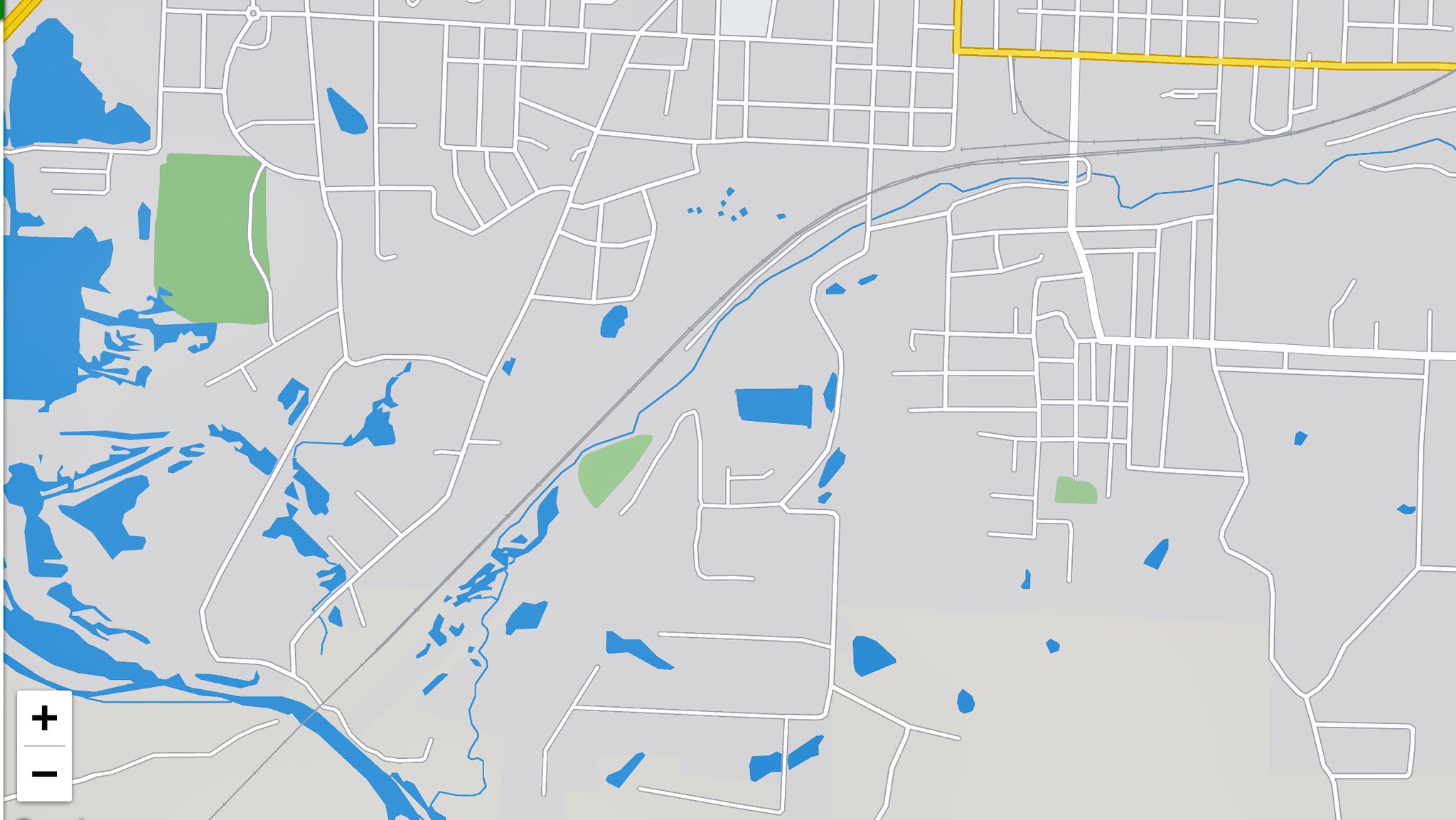A digital map serves as the focal point of this image, characterized by its predominantly grey color scheme. Any bodies of water are highlighted in subtle blue tones. The map itself is quite basic, depicted as a skeleton framework with roads rendered in simple white lines. Most of the notable features are located on the left-hand side, where several large patches of blue indicate water inlets and rivers. Additionally, there is a prominent green square representing a playing field. The road layout forms an intricate pattern across the map, but lacks detailed information. At the bottom of the image, a plus and minus sign are present, providing zoom functionality. Currently, there are no labels or names on the map, but it is implied that further details such as road names and landmarks may appear upon zooming in.